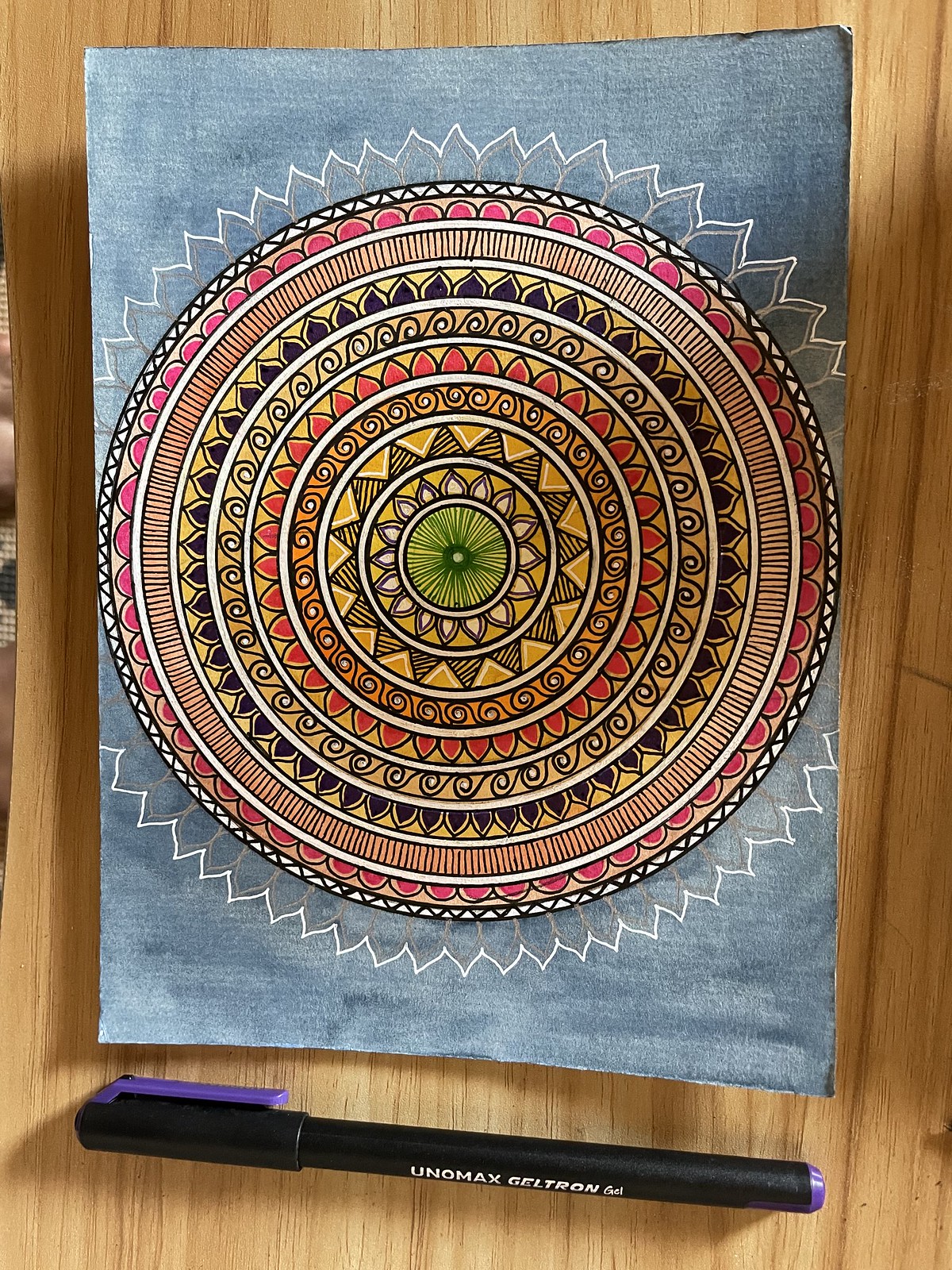This portrait-mode image features a detailed setup on a light brown, wooden table characterized by darker vertical stripes running from top to bottom. On the table, a black gel pen is prominently placed diagonally from the bottom left to the bottom right. The pen is identified as a UNOMAX GELTRON gel pen, with distinctive purple accents on the right side, including the cap and a latch for pocket attachment.

Above the pen lies an artistically intricate design, presumably created using gel pens. The artwork initiates from a central green dot, expanding outward in a series of elaborately detailed layers. The central dot is encircled by dark green, followed by radiating green rays, a white stripe, and a series of pointed petals that might be trimmed in purple. Continuing outward, the design includes a white circle, black-striped triangles, another white circle, black waves with small white dots, more white circles, rounded reddish petals, light yellow waves, and black petals outlined in black, each section separated by white circles.

The pattern further extends outward with black stripes, pink half-circles outlined in black, and a concluding black circle. The entire design is framed with light gray and white petals, set against a gray background on paper. This intricate piece complements the simplicity of the wooden table and the lone black pen, creating a harmonious and visually captivating composition.